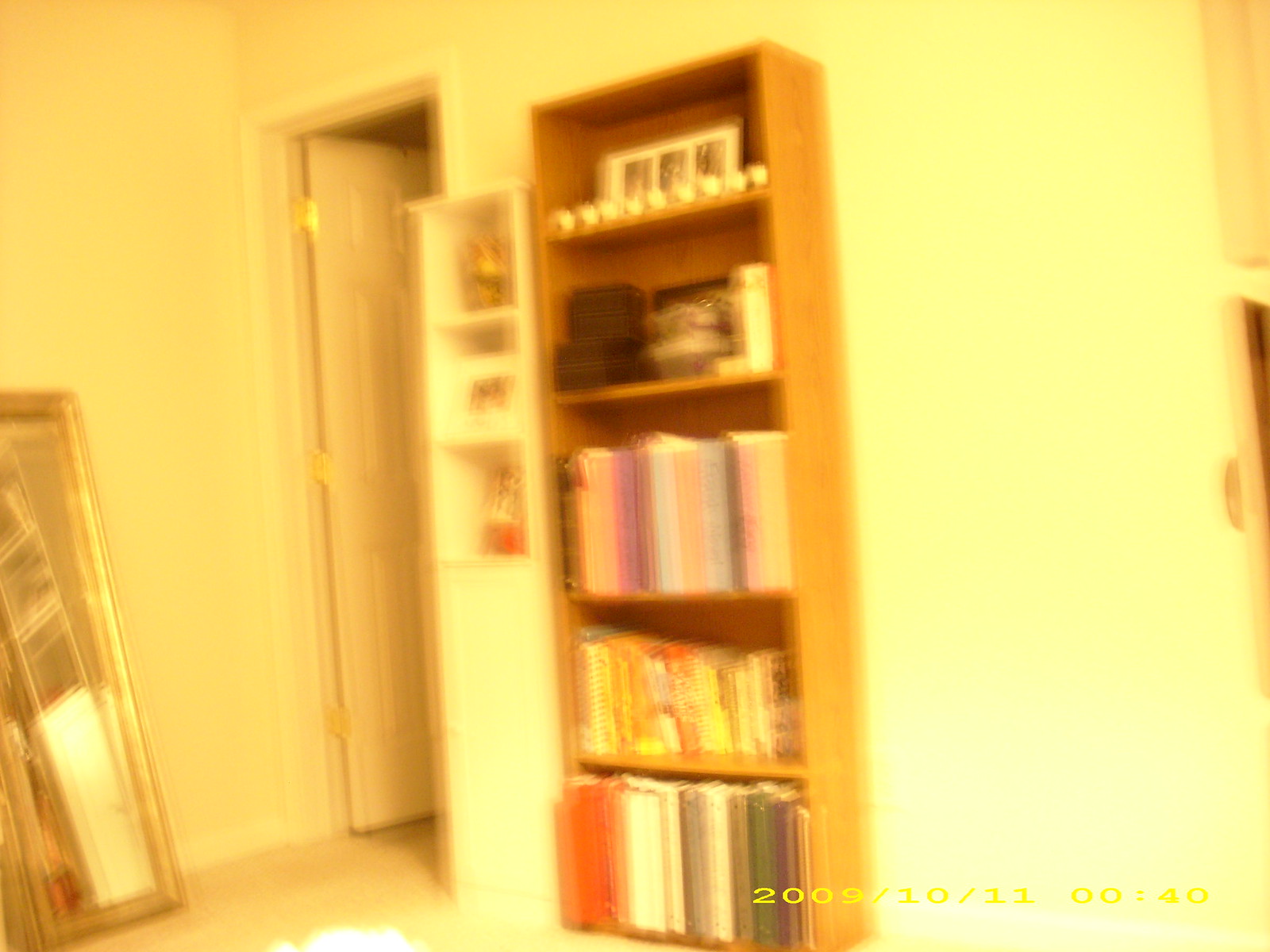This dated and slightly hazy photograph, marked with the timestamp "2009/10/11 00:40" in the bottom right corner, appears to depict an interior room with strong yellow walls, likely due to poor color balance. The focal point is a five-tier light tan wood bookshelf, positioned to the right of a white door with gold-colored hinges, which opens outward into a dark space, possibly a closet or hallway. The top two shelves of the bookshelf hold various items, including boxes and candles, while the bottom three shelves contain an assortment of colorful books whose details are indiscernible. Adjacent to the bookshelf, there is a narrower white cabinet-style bookcase displaying decor and pictures, though the contents are blurred. Leaning against the wall, near the white doorframe, is a long rectangular mirror, adding to the room's eclectic decor.